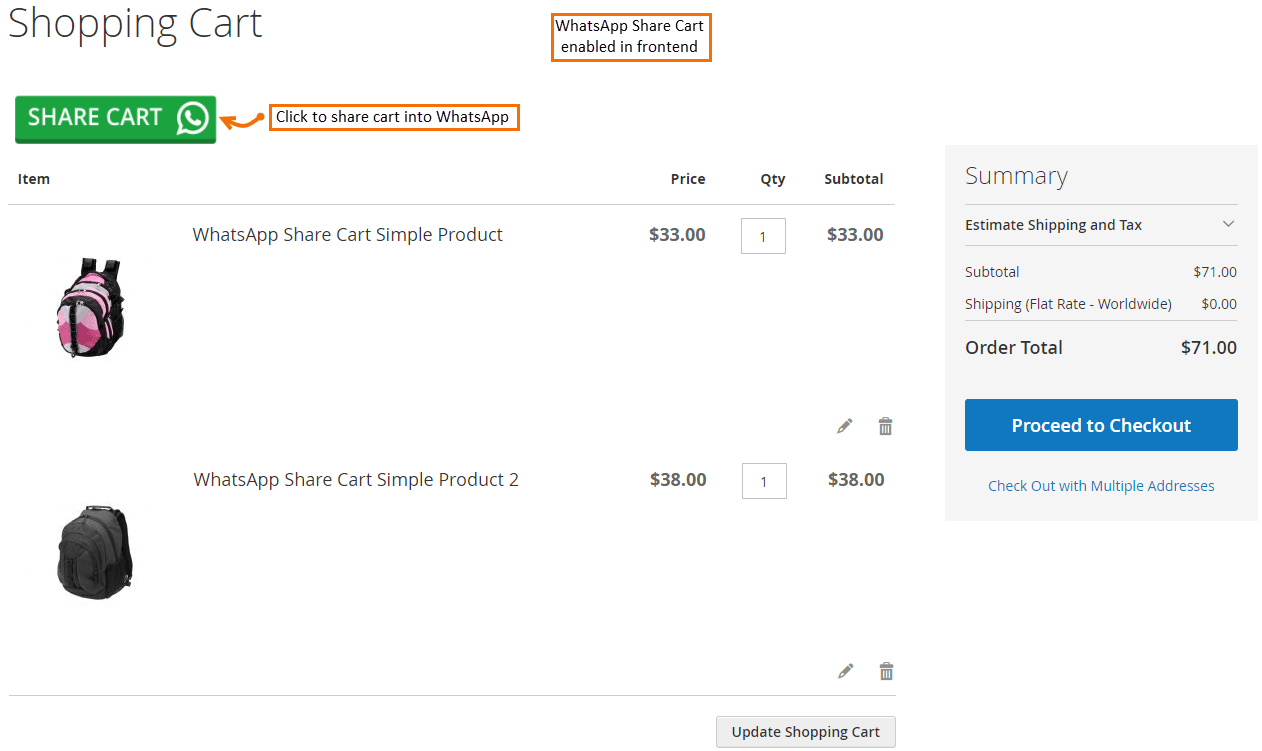This is a screenshot of a "WhatsApp Share Cart" interface on a shopping website. At the top left corner, there is a label that reads "Shopping Cart." Directly below it is a green button labeled "Share Cart," accompanied by an icon resembling a phone handle. An arrow pointing towards this button bears the text "Click to share cart into WhatsApp," all outlined within a red rectangular box. To the right of this section, there is another red box containing the text "WhatsApp Share Cart Enable Front End."

Below this header section, a list of items in the cart is displayed. The first item is an image of a backpack with the label "WhatsApp Share Cart Simple Product." It is priced at $33 with a quantity of one, leading to a subtotal of $33. The second item is another backpack, labeled "WhatsApp Share Cart Simple Product 2," priced at $38 with a quantity of one, but its subtotal is incorrectly listed as $33. Both items feature "Edit" and "Trash" buttons that allow the user to modify or delete the items.

On the right side, there is a summary section outlined in a smaller rectangle. This section includes "Summary," "Estimated Shipping and Tax" as a dropdown menu, "Subtotal: $71," and "Shipping: Flat Rate Worldwide ($0)." The "Order Total" is listed as $71.

At the bottom of the summary section, there is a prominent blue button labeled "Proceed to Checkout," and beneath that, a blue link that reads "Checkout with Multiple Addresses."